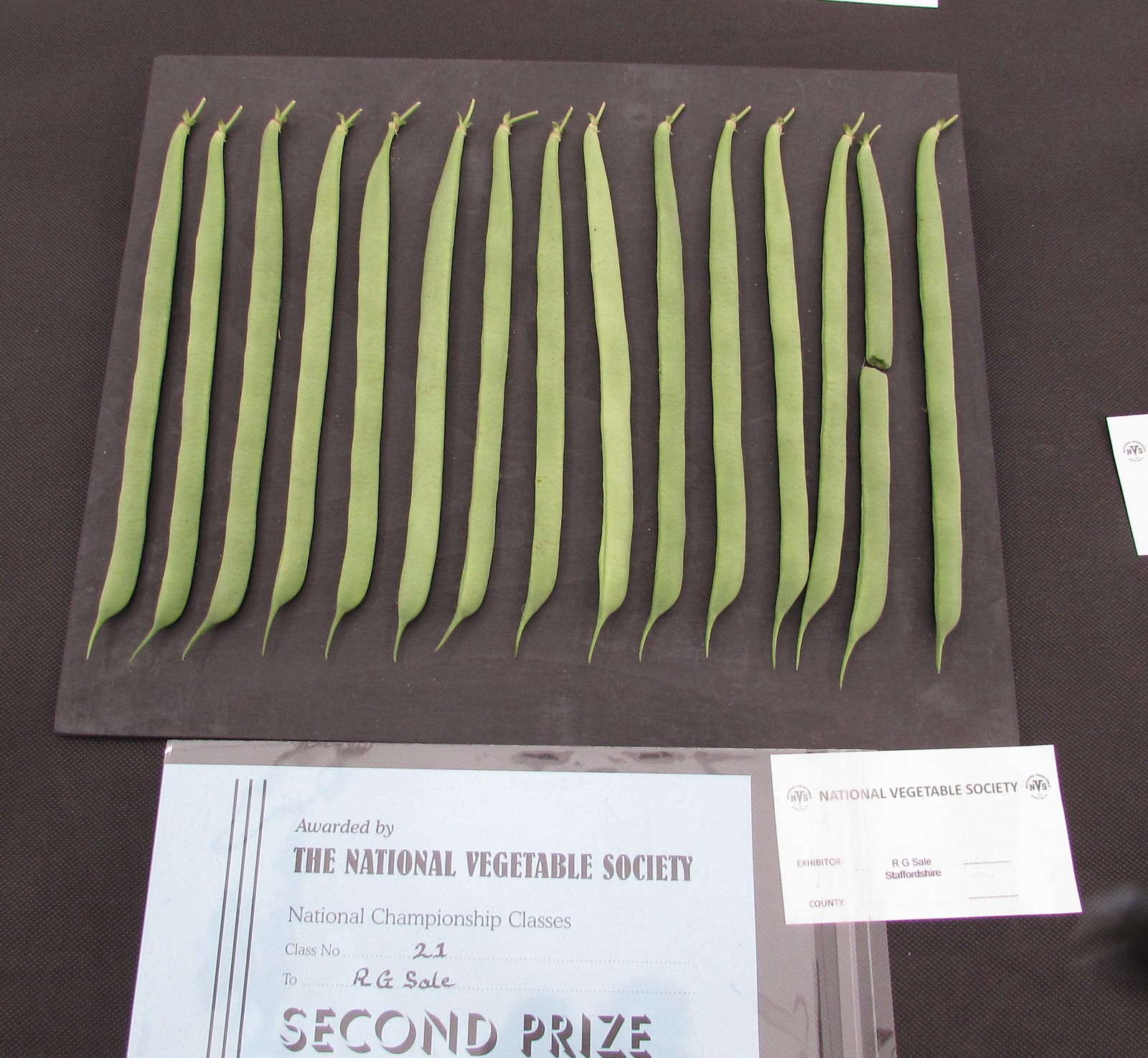The image depicts a vertical, rectangular photo with a black background. Positioned on a black napkin in the top two-thirds of the frame are 15 meticulously arranged green string beans, one of which is slightly cracked on the right-hand side. These vibrant green beans have earned recognition in a string bean contest. In the bottom third of the image, a blue paper card proudly announces that the beans have been awarded second prize by the National Vegetable Society in the National Championship classes, specifically class number 21, and it is made out to an exhibitor named RG Sale. Adjacent to the prize card is a small white business card also bearing the name of the National Vegetable Society and spaces labeled for the exhibitor and county. The entire setup is displayed on a brown table, highlighting the exceptional quality of the beans that secured the coveted second prize.